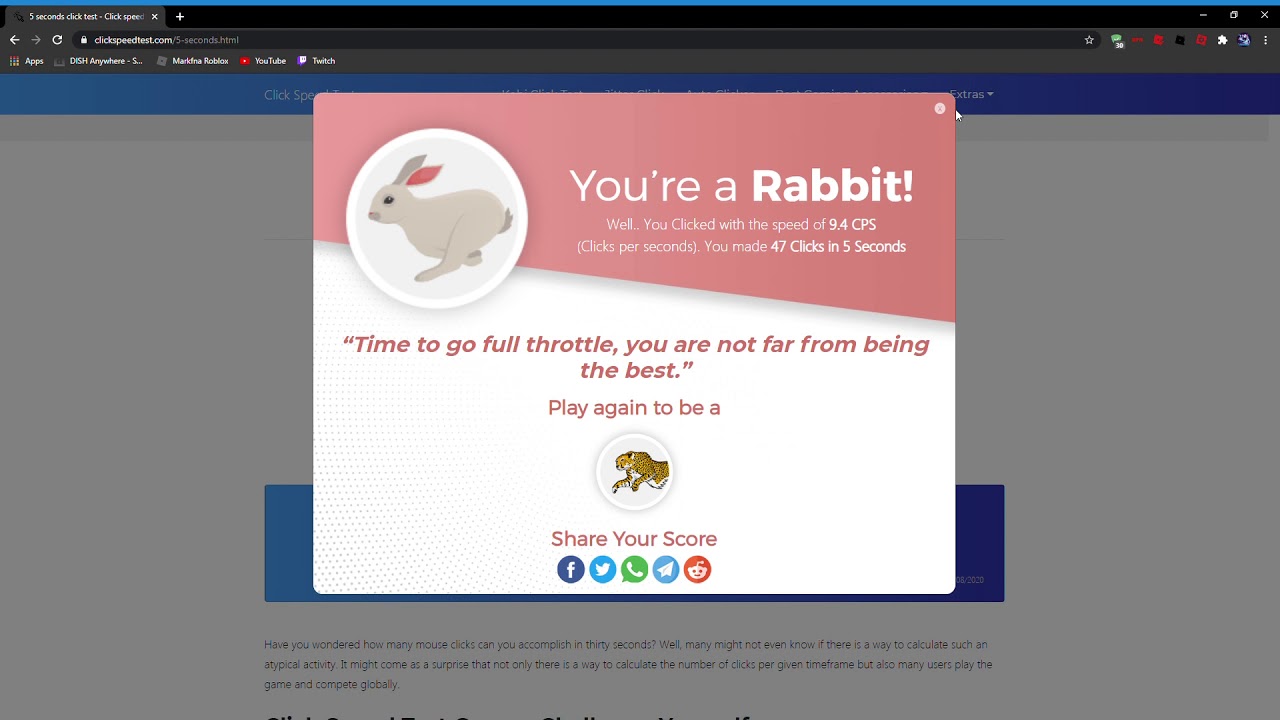The image showcases a browser window with a black border at the top. One tab is open, which displays the heading "5 Second Click Test - Click Speed." Nearby, a white 'X' icon allows users to close the tab, and a white '+' sign enables the addition of new tabs. Below this, a white arrow points left, beside a light gray URL that reads "clickspeedtest.com/5-seconds.html."

The background is gray due to an active pop-up window. This pop-up is rectangular, with its top portion colored light red and the bottom white. On the left side of the pop-up, there's a white circle containing a grayish bunny rabbit graphic. To the right of the circle, text reads: "You're a rabbit! You clicked with a speed of 9.4 CPS (clicks per second). You made 47 clicks in 5 seconds."

Further down, in reddish font on a white background, the message encourages the user: "Time to go full throttle. You are not far from being the best. Play again to be a cheetah." Below this, icons for sharing the score on Facebook, Twitter, and WhatsApp are displayed, with an additional unidentified blue and reddish icon.